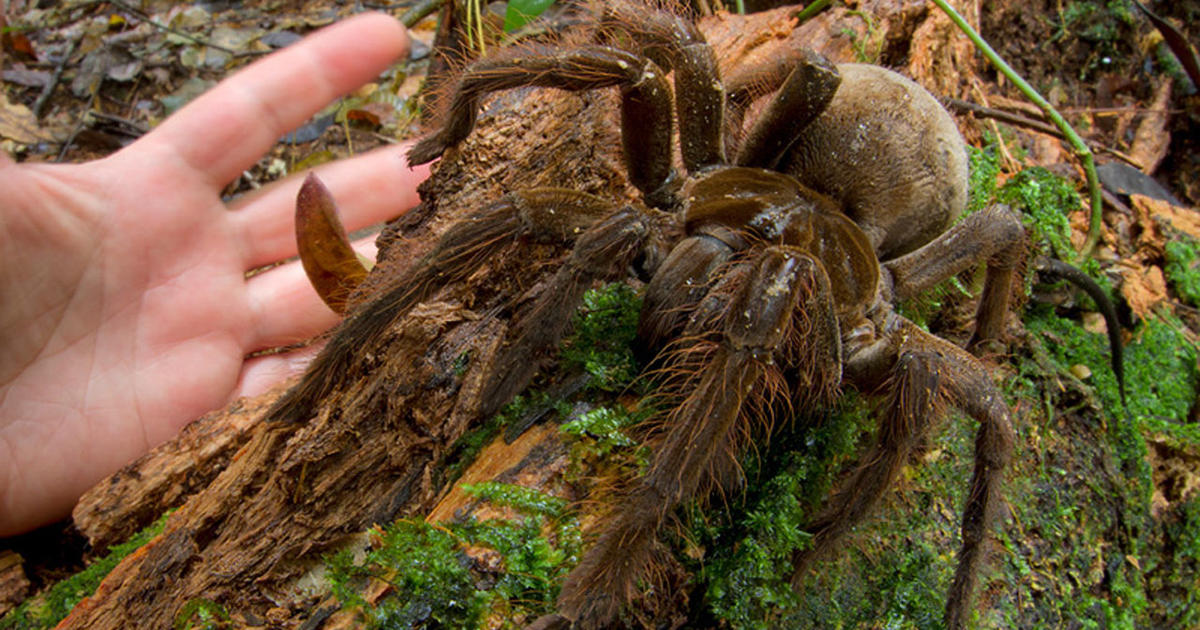The photograph, taken outdoors, captures a massive dark brown spider perched on a moss-covered log. The spider, which appears larger than a human hand positioned on the left for scale, is facing towards the viewer with its front legs slightly raised. The spider's body is divided into a lighter round abdomen and darker, hairy legs, equipped with visible, menacing fangs. The setting seems to be a forest floor, characterized by moist, rain-soaked ground, scattered dead leaves, and additional vegetation visible in the background. The log it straddles is lighter brown, adding to the rustic, natural ambiance of the scene.